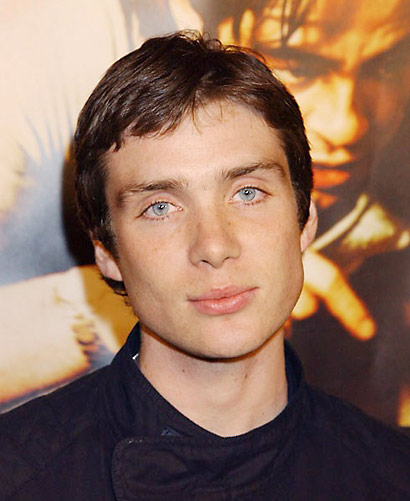This photograph depicts a close-up headshot of a young Cillian Murphy, likely in his 20s. The image shows him from the neck or shoulders up. Cillian Murphy has pale skin, deep blue eyes (mistakable for light hazel or gray), and medium-length brown hair parted to the side. He has medium bushy eyebrows and is completely clean-shaven. His head is slightly tilted to the left, and he wears a black jacket or shirt. Cillian presents a subtle smirk while looking straight at the camera. In the background, there is a movie poster featuring another young person with longer hair, who appears to be looking to the side and holding something, although the details are not very clear.